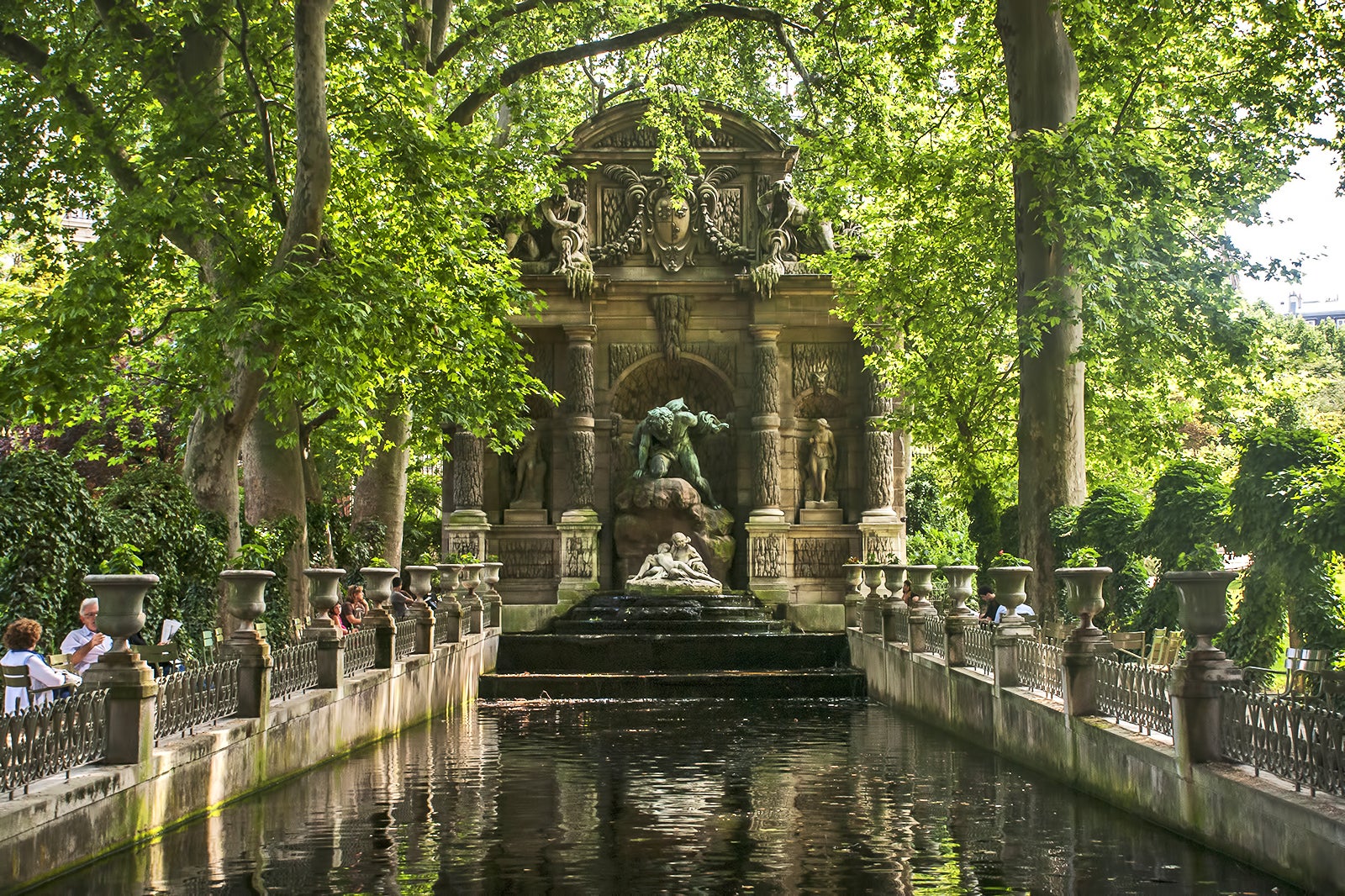This photograph captures an enchanting outdoor scene, possibly in a park, with a grand stone fountain as the centerpiece at the end of a small canal, which feels like a concrete river. The tremendous central fountain features a greenish, likely bronze figure of a man bending down on a rock, now aged to a verdant patina. Flanking the central figure are two smaller childlike figures, while higher up, two statues of women in dresses and hats are carved into the fountain, facing the centerpiece. Above these, two additional statues kneel, holding amphorae from which stone-carved liquid appears to pour. 

The water from the fountain cascades down four black steps, flowing towards the viewer along the canal. On either side of this canal are stone walls adorned with fencing, which is punctuated by regularly placed urns or flower pots brimming with plants. Just beyond the fencing, areas are set up for dining, where people are seen enjoying meals, sitting, observing the beautiful scenery, or engaging in conversation. The canal and dining areas are shaded by draping trees and lush landscaping, creating an inviting atmosphere. The entire scene is overhung by abundant foliage, including ivy and numerous shade trees, adding to the tranquil and enticing ambiance of this charming outdoor setting.